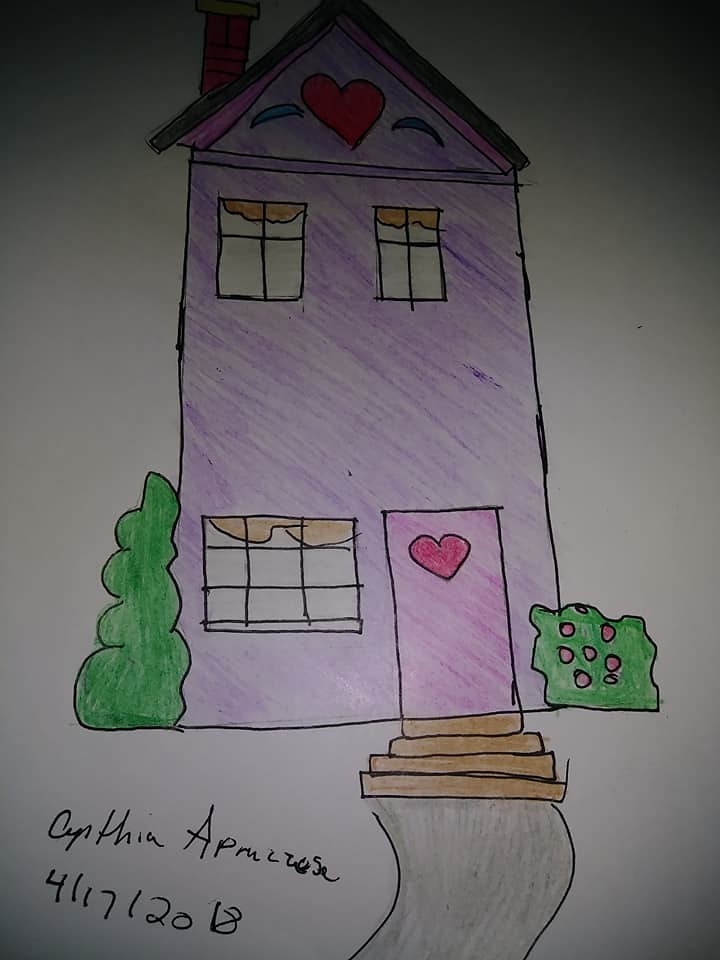This hand-drawn illustration on plain paper showcases a narrow and tall purple house, crafted with a marker and colored in with crayon. The house features charming details like a heart on the very top of its roof. The top floor boasts two windows, while the bottom floor has one large window and a pink door adorned with a pink heart. Brown steps lead down from the door to a gray walkway. Adding to the scene, there is a green tree on the left side of the house and a green bush on the right. The artist, Cynthia A., has signed the drawing in the bottom left corner along with the date, 4-17-2018.